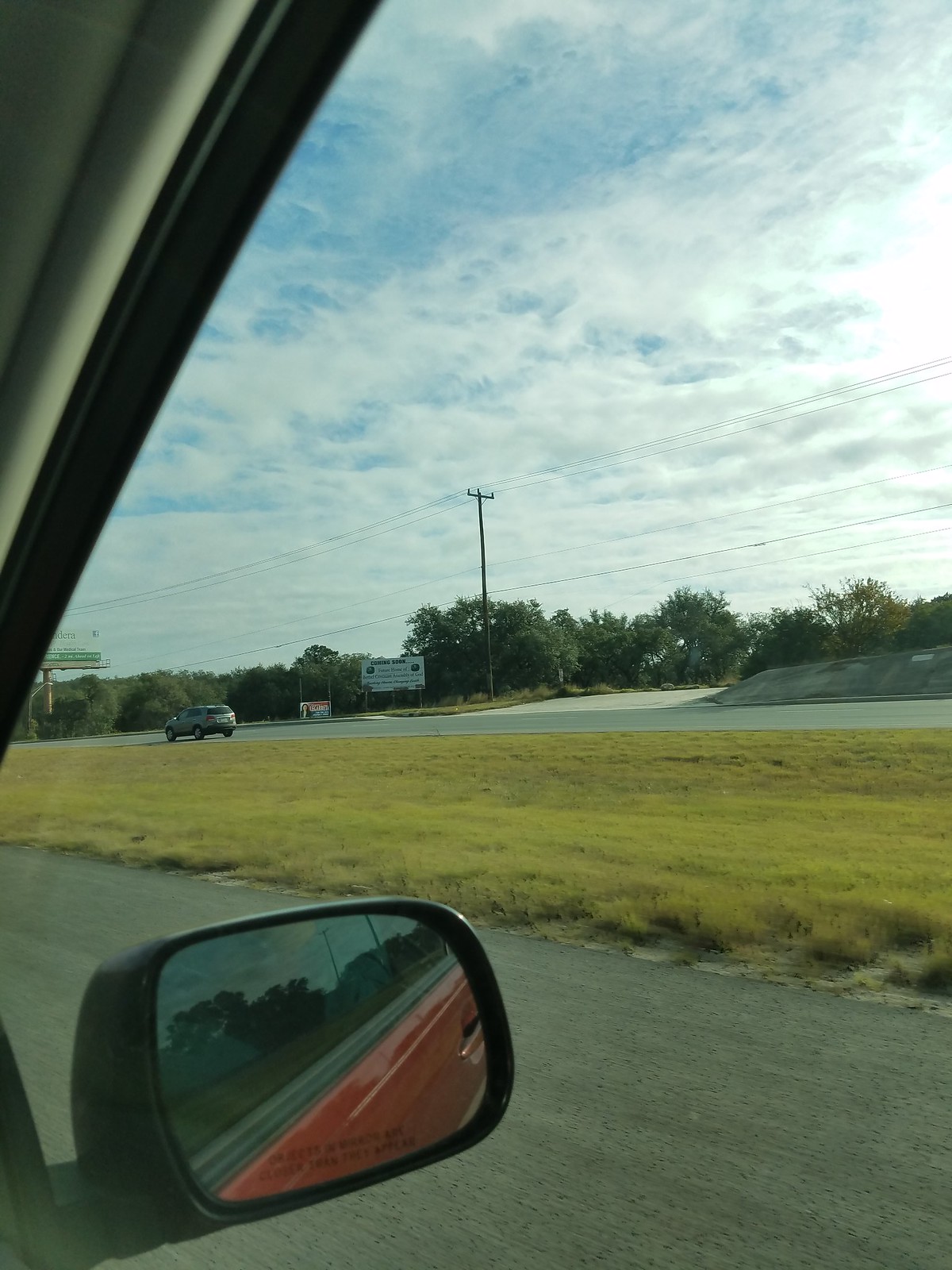In this photograph taken from the passenger side window of a vehicle, likely a dark red car, we see the exterior side mirror and a part of the car’s frame reflecting in the mirror. The car appears to be either driving on or pulled off to the side of a dirt road. A grassy median separates this vehicle from a gray SUV driving along on another road further away. The background is filled with lush trees beneath a blue sky dotted with clouds, and a few billboards, although the text on them isn't visible. The composition suggests a scene of casual travel on a semi-rural route.